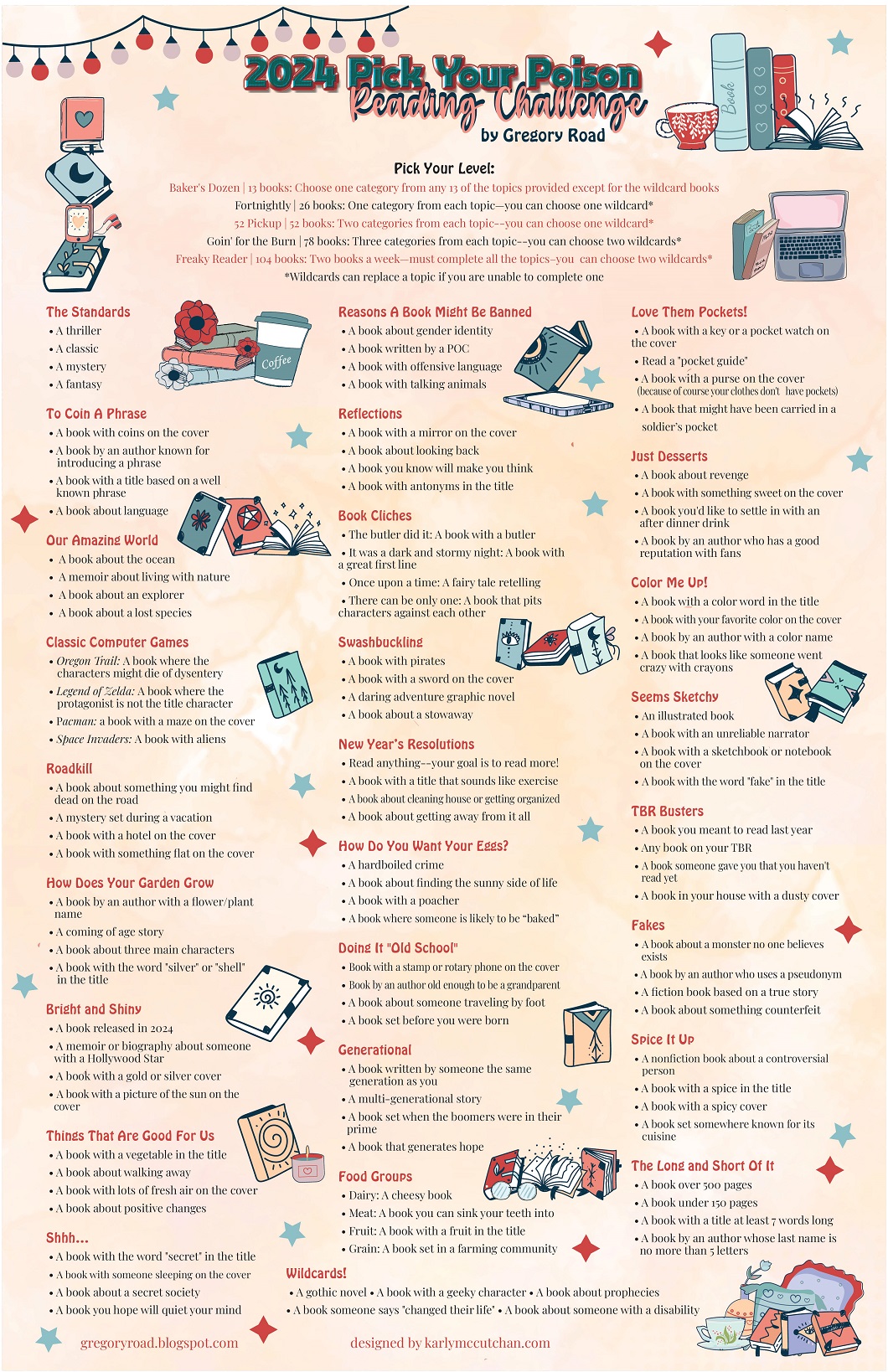"2024 Pick Your Poison Reading Challenge Flyer: A vibrant, single-page flyer with a salmon and light pink background adorned with whimsical illustrations in blue, red, dark blue, white, and black. At the top, a charming garland of lanterns hangs across, setting a festive tone. The bold title '2024 Pick Your Poison Reading Challenge' is prominently displayed, attributed to Gregory Road or Rand. Accompanying this, a delightful illustration features a collection of hardback books, with one lying open beside a teacup, inviting readers to embark on a literary journey.

Below the title, the phrase 'Pick Your List' encourages participants to choose from a diverse array of book types, although the small font headers in red are difficult to decipher. Multiple small illustrations scatter the page, depicting stacks of books, some embellished with flowers or partnered with takeout coffee cups, as well as books in various positions—both flat and upright. Despite the tiny, challenging-to-read text, the flyer presents an enticing and meticulously designed reading challenge, sure to captivate any booklover."